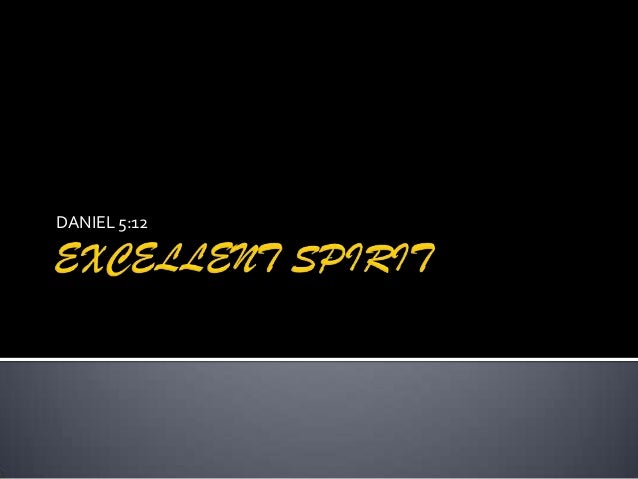This image resembles a presentation slide and features a stark, minimalist design. The background is predominantly black, occupying about 75% of the space, while the remaining 25% at the bottom is grey with a subtle gradient, darker at the edges and lighter toward the center. A small, horizontal white line separates these two sections. Centrally positioned on the black background is the text "Daniel 512" in small white font, indicating a biblical reference. Directly beneath it, in large yellow cursive, is the phrase "Excellent Spirit," with the distinct and stylistic detail where the Ts resemble the number seven.